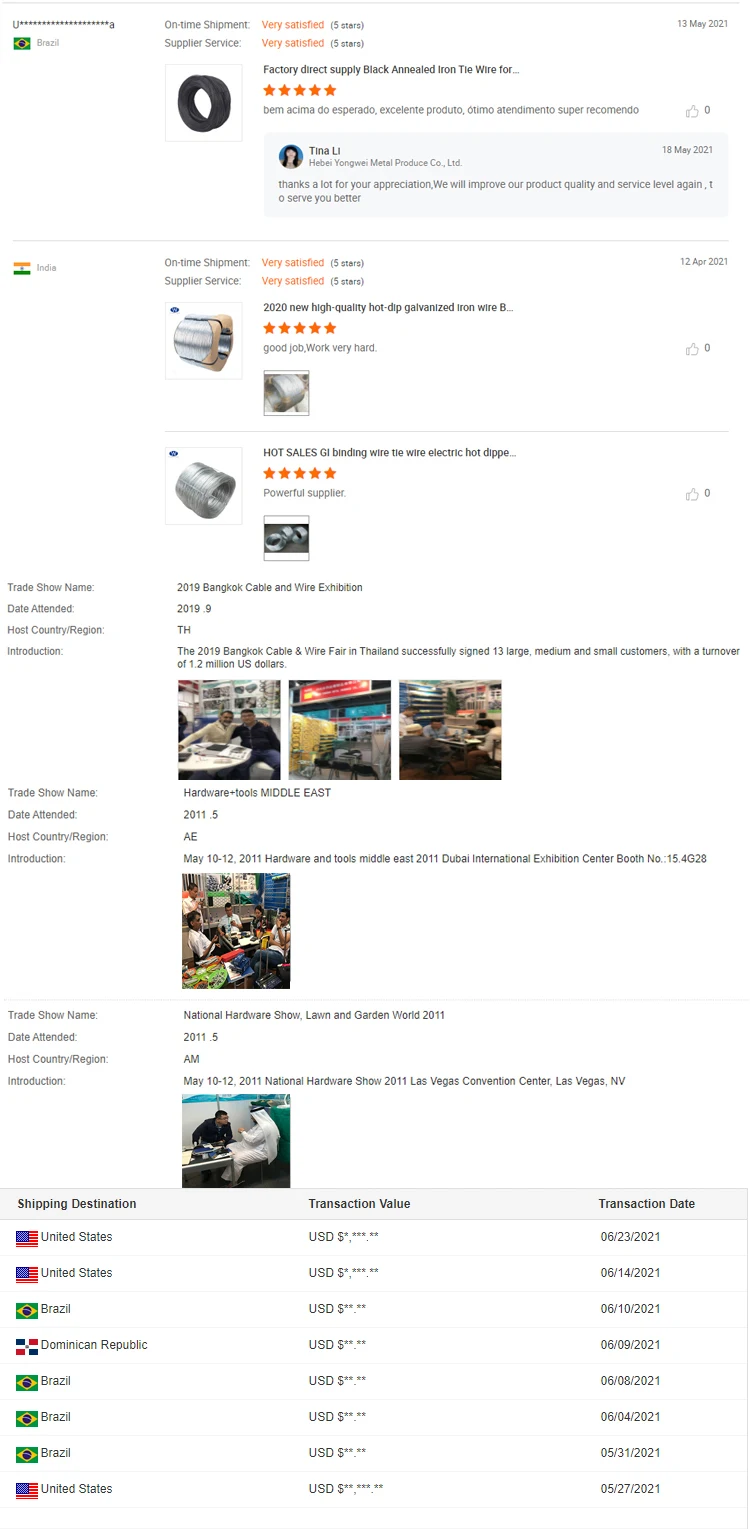This is a detailed caption for the image:

---

A screenshot of a smartphone screen showcasing a shopping app interface. At the top, multiple columns display various items available for purchase. The highlighted product at the top is labeled, "Factory Direct Supply Black Annealed Iron Tie Wire," with the title truncated by an ellipsis. This product boasts a five-star rating. A customer review is visible beneath the product listing, stating, "Thanks a lot for your appreciation. We will improve our product quality and service level again to serve you better."

Further down, more products are listed, including one with the label "On-time Shipment," featuring a high-quality hot-dip galvanized wire. Another item, titled "Hot Sales GI Binding Wire," has its description partially cut off, showing the words "the wire electric" and "hot dipped." As the page scrolls, it reveals images of people using these items in various contexts. The top section showcases three images, while the subsequent sections each display a single image.